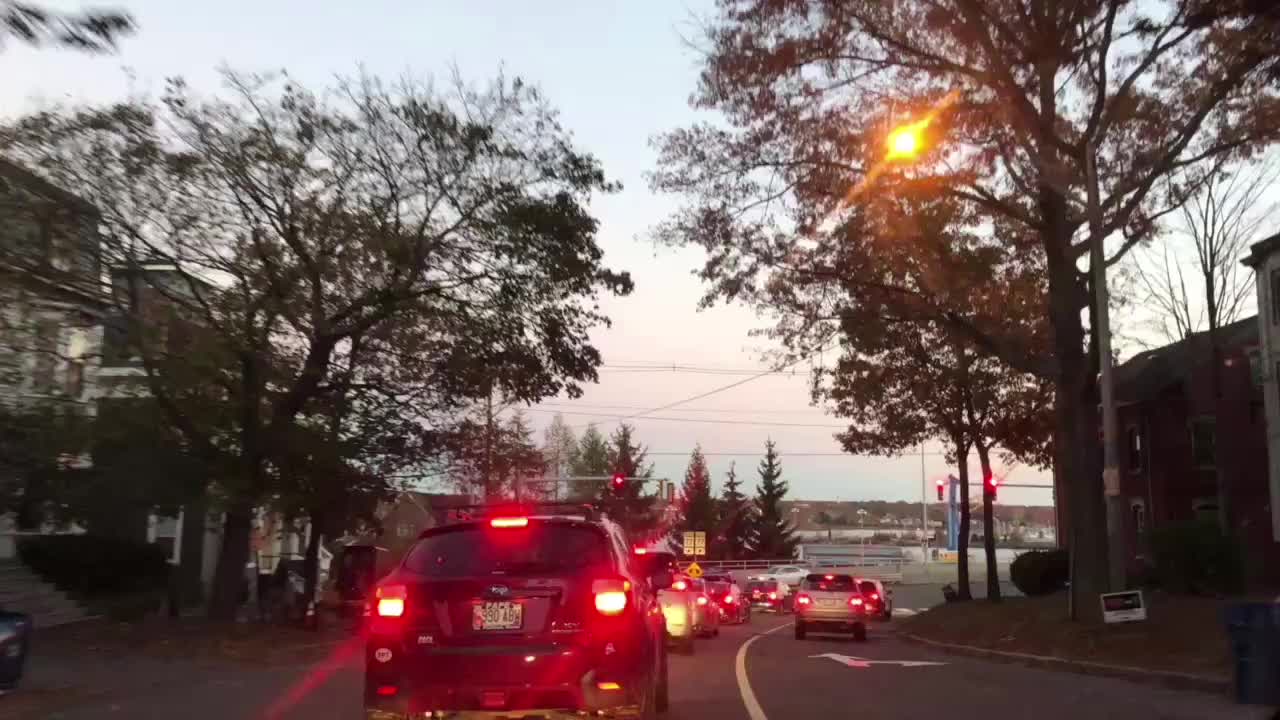This image captures a serene one-way street with two lanes lined with cars at a standstill, awaiting the change of the red traffic light visible in the distant background. Spindly trees with sparse foliage border both sides of the street, adding a touch of greenery. To the left, quaint houses nestle behind the trees, with pathways leading to their entrances; one building, distinguished by an elongated white window, might be a shop. On the right-hand lane, behind the last car in line, a signpost indicates directions for motorists to either continue straight or make a right turn. The overall scene is calm, with the setting sun casting a warm glow, highlighting the urban tranquility.